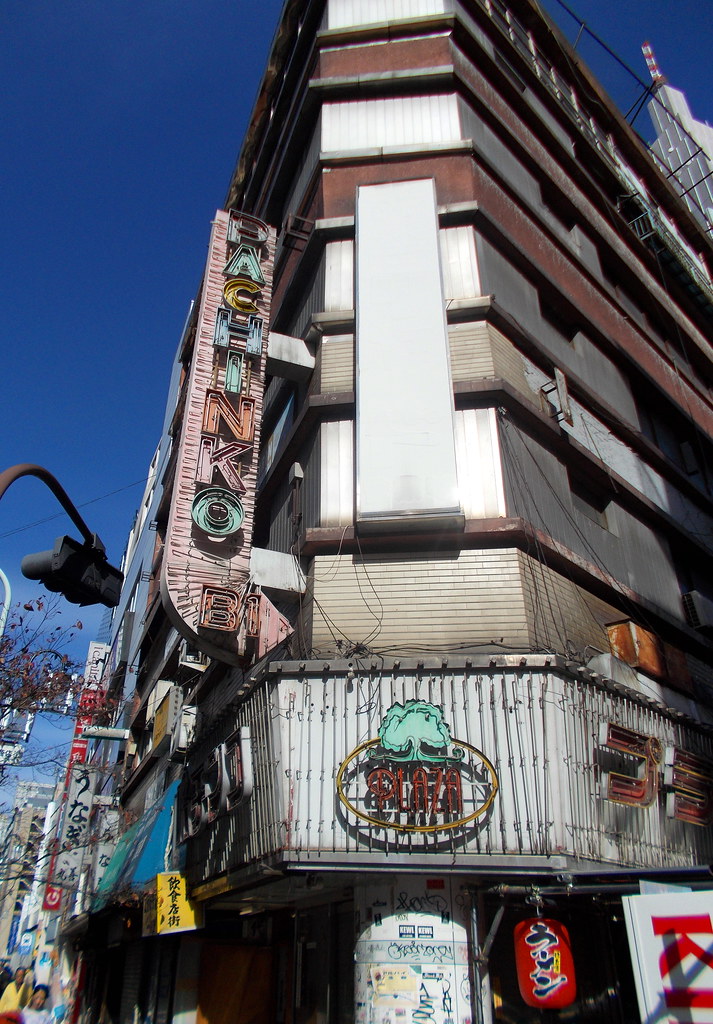This detailed, color photograph, taken in portrait orientation, captures the facade of a large, multi-story building at the corner of intersecting streets in what is likely the Shinkai district in Tokyo, Japan. The building, a mix of white sections and brick with recessed balconies, features a prominent vertical sign on its left side that reads "Pachinko" in multiple colors, likely neon-lit at night. The sign also includes an arrow pointing toward the building entrance. The scene, set against a crystal blue sky without a cloud in sight, includes several other Asian-script signs and neon features, indicative of an area full of vibrant nightlife. At the base of the building, there is a canopy with oval-shaped signage in red lettering, and a traditional red lantern with black kanji characters hangs nearby. The sidewalks showcase the lively street life, with pedestrians walking by, a brown tree, and a streetlight or traffic signal partially visible on the left. Other nearby buildings feature similarly styled signs, reinforcing the bustling urban atmosphere.